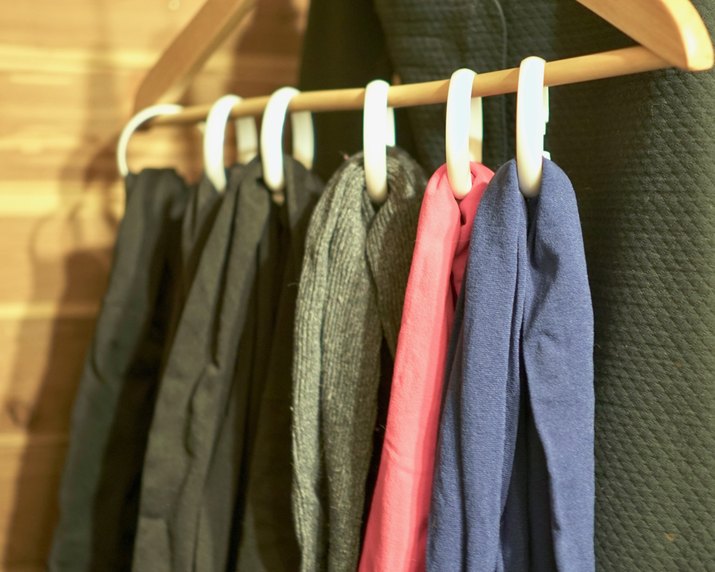In this flash photograph, a large wooden hanger with a sleek, thin bar spanning across its width is prominently displayed. Known for its sturdiness and weight, this hanger is partially cut off at its top by the frame, with the bottom gear hanging at the upper section of the image.

Suspended from the hanger's bar are six metal or possibly plastic rings, their precise material indistinguishable due to the intense glare from the flash. Each ring supports a scarf, with the collection presenting a variety of textures and colors. The scarf furthest to the right appears to be made of blue terry cloth, while the adjacent one boasts a sheer, pink fabric. Next in line is a gray, ribbed scarf, and the final three, slightly blurred, seem to be black.

These scarves cast shadows on the wooden planks behind them, suggesting they may be hung in a cedar closet. Adding to the scene's diversity, the right side of the image reveals the textured presence of a black cotton suit jacket, hinting at a well-organized wardrobe.